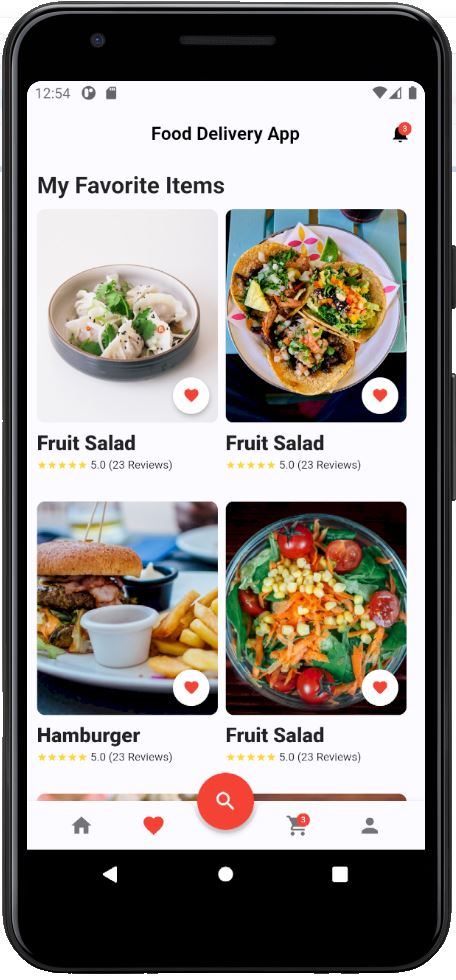The photograph displays a black cell phone set against a white background, showcasing the device's side buttons. The phone screen exhibits various details and app icons. In the upper left corner, the time reads 12:54, and an unidentified icon is nearby. On the upper right, there are indicators for Wi-Fi connectivity, cell signal strength, and a fully charged battery.

The center of the screen prominently features a "Food Delivery App" display. To the right of this title, there is a bell icon with a red circle containing the number three, indicating notifications. Below the title, the section labeled "My Favorite Items" lists four food items in two rows.

The first row consists of:
- Left: "Fruit Salad, five stars, 23 reviews" (accompanied by an image of Chinese dumplings)
- Right: "Fruit Salad, five stars, 23 reviews" (with an image of tacos)

The second row displays:
- Left: "Hamburger, five stars, 23 reviews" (the only accurately depicted item)
- Right: "Fruit Salad, five stars, 23 reviews" (illustrated with a salad image)

At the bottom center of the screen, there is a red circle with a white magnifying glass icon, representing the search function. Beneath this, a navigation bar includes four icons from left to right: a home icon, a heart, a shopping basket (with a red circle indicating three items), and a person icon.

The image ironically highlights that despite the labels indicating "Fruit Salad," the visual content for three out of the four items is incorrect, depicting Chinese dumplings, tacos, and a salad instead. The only correctly labeled image is the hamburger.